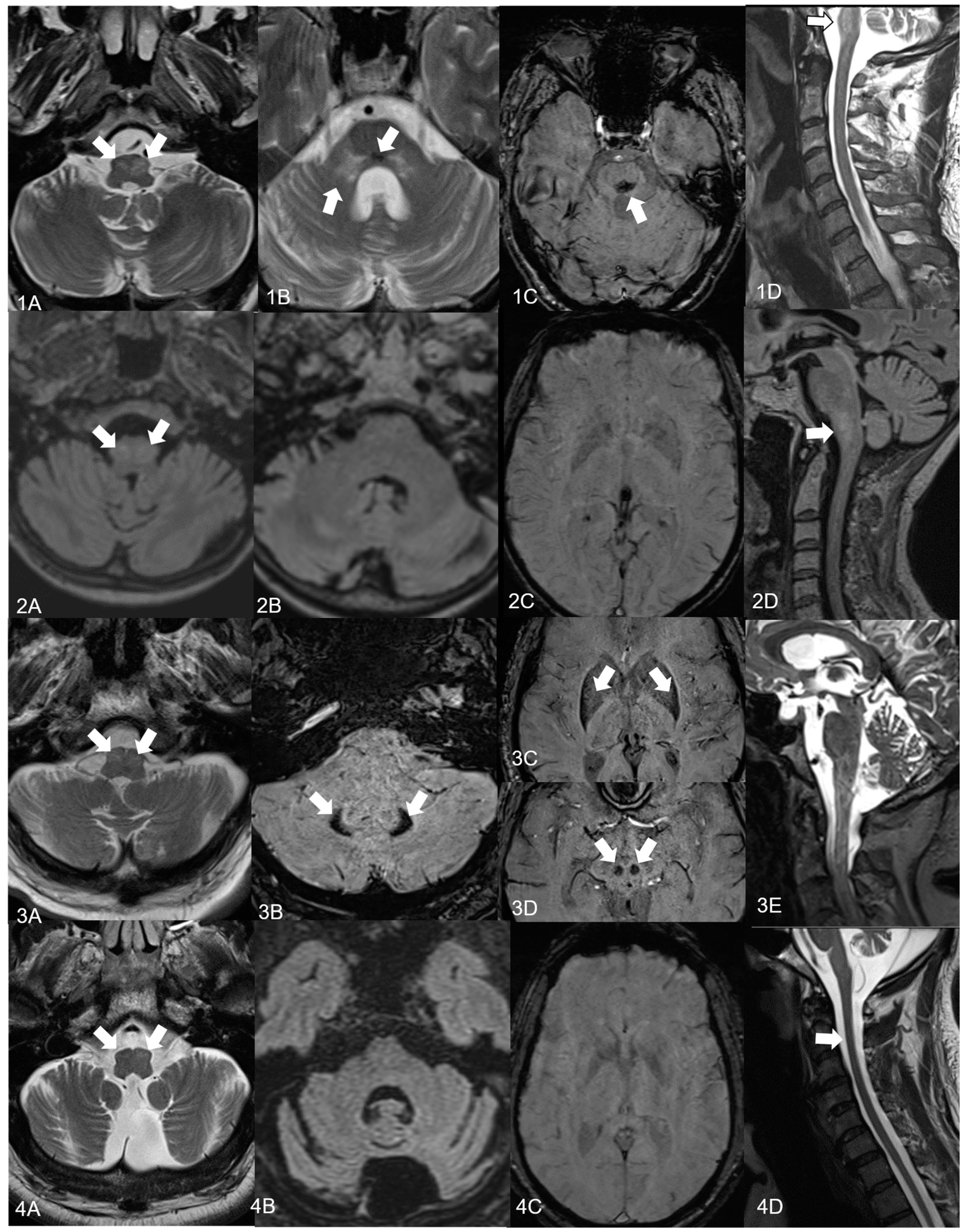This image is a detailed monochrome photograph showcasing multiple brain scans organized in a 4x4 grid. Each panel is labeled sequentially from 1A to 4D, creating four rows and four columns. The first row includes images labeled 1A, 1B, 1C, and 1D; the second row consists of 2A, 2B, 2C, and 2D; the third row contains 3A, 3B, 3C alongside 3D stacked vertically, and 3E; the fourth row follows with 4A, 4B, 4C, and 4D. Each brain scan presents different cross-sectional views in shades of black, white, and gray, with a consistent black background. The scans indicate various layers and lobes of the brain, with column D focusing on the spinal cord's connection to the brain. White arrows are noted throughout the panels, pointing to specific anatomical features or potential findings, directing attention to areas of interest. This collection of images serves to highlight different anatomical orientations and structural details visible in either MRI or CT scans. The consistent and detailed labeling enhances the comprehension of each panel's specific focus within the grid layout.